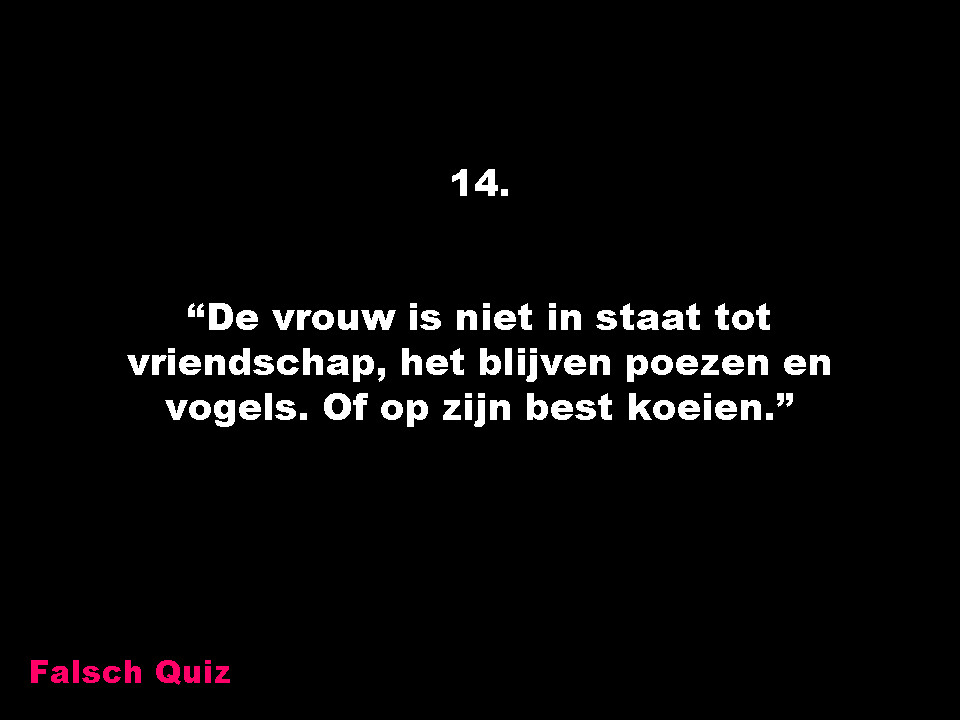The image features a solid black background with text prominently displayed in the center. The text consists of three lines written in what appears to be German, making it unreadable for those not familiar with the language. It reads: "D-E V-R-O-U-W I-S N-I-E-T N-S-T-A-A-T T-O-T, V-R-I-E-N-D-S-C-H-A-P, H-E-T B-L-I-J-V-E-N P-O-E-Z-E-N E-N, V-O-G-E-L-S. O-F O-P Z-I-J-N B-E-S-T K-O-E-I-E-N." Above this text, the number "14." is centered at the top. In the bottom left corner, the text "Falsch quiz," which translates to "False quiz" in English, is written in pink letters. The image gives the impression of a classroom or educational setting, perhaps used by a teacher to present a quote for students to memorize, potentially for an upcoming exam or social media post styled as an informative slide. The colors in the image are primarily black, white, and purple.